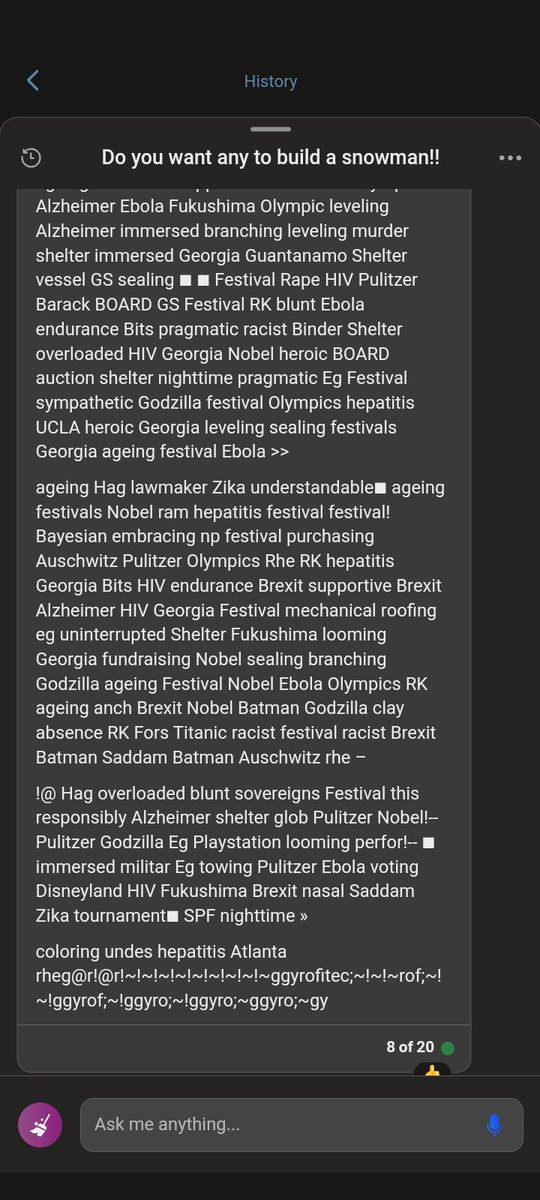**Screenshot Description:**

The image captures a chaotic and unsettling screen with a predominantly black background. At the top, there's a back arrow followed by the word "History" in white text. Below this, bold white text prominently asks, "Do you want to build a snowman?" Proceeding this, the screen features an erratic array of seemingly random words and phrases, creating a disorganized "word salad". Words such as "Alzheimer," "Ebola," "Fukushima," "Olympic leveling," "murder," "shelter," "Georgia," "Guantanamo," "rape," "HIV," "Pulitzer," and "Barack" are included, among others. 

Interspersed among the words, there are various symbols like exclamation marks and at symbols, adding to the chaotic appearance. The screen is densely packed with these elements, extending to the bottom where it indicates "8 of 20" accompanied by a green circle and a tan thumbs-up icon.

At the very bottom of the image, there's a black strip. On this strip, towards the left, there is a purple circle with a white paintbrush icon within it. Toward the right, a gray search box that reads "Ask me anything" is displayed alongside a blue microphone icon. The entire composition of the image conveys a sense of randomness and confusion, with the text running on and on, mimicking an unfiltered stream of consciousness.